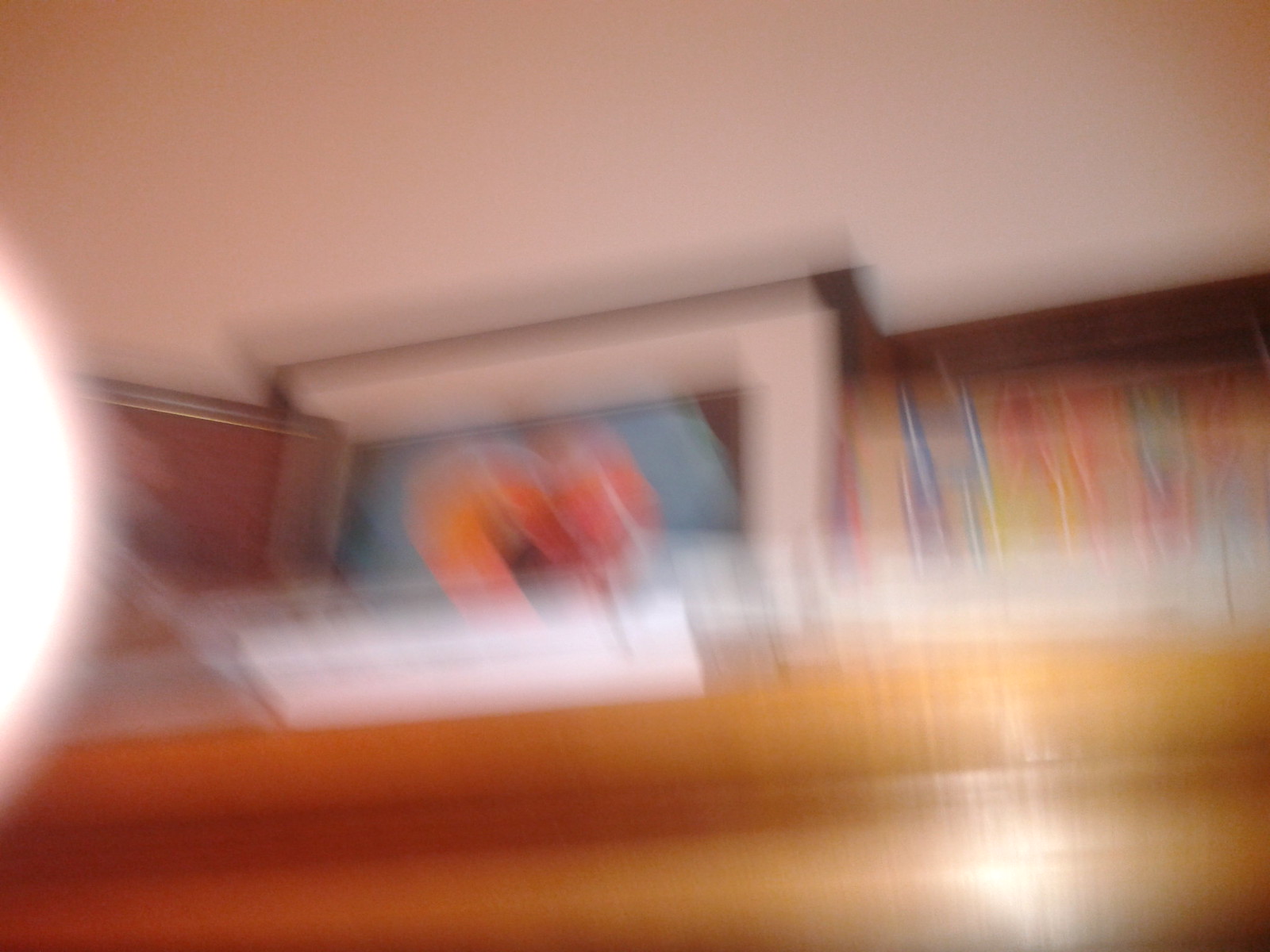The image is likely taken in motion, resulting in a noticeable blur. It depicts a wooden surface, possibly a shelf or table, upon which three picture frames are standing upright and closely grouped together. All the frames are brown in color but contain different pictures inside. The central frame features a photo with a white border and a dominant red heart set against a blue background. The two flanking frames are significantly blurry, displaying predominantly reddish hues. On the far left edge of the image, a bright, white object resembling a finger is visible. The background includes a white wall, contributing to the overall illumination of the scene.